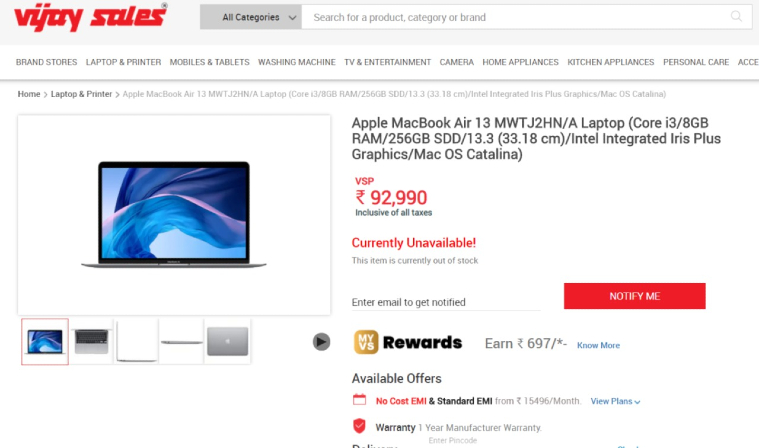**Image Caption:**
The website appears to be dedicated to tech sales, specifically under the brand name "VIJAY Sales" (alternatively spelled V-U-G-A-Y or possibly written in a non-English script with diacritical marks). The featured product is an Apple MacBook Air 13, model MWTG2HN/A. 

- **Product Specifications:**
  - Processor: Core i3
  - Memory: 8GB RAM
  - Storage: 256GB SSD
  - Display: 13.3-inch (33.18 cm) screen
  - Graphics: Intel Integrated Iris Plus
  - Operating System: Mac OS Catalina

- **Pricing and Availability:**
  - Price: 92,999 VSP (inclusive of all taxes)
  - Availability: Currently unavailable, with a notification option for restocking

- **Reward Details:**
  - Earns: 697 VS Rewards points with the purchase

The visual depiction includes a main image of the MacBook Air 13, accompanied by five additional images showcasing the laptop from various angles.